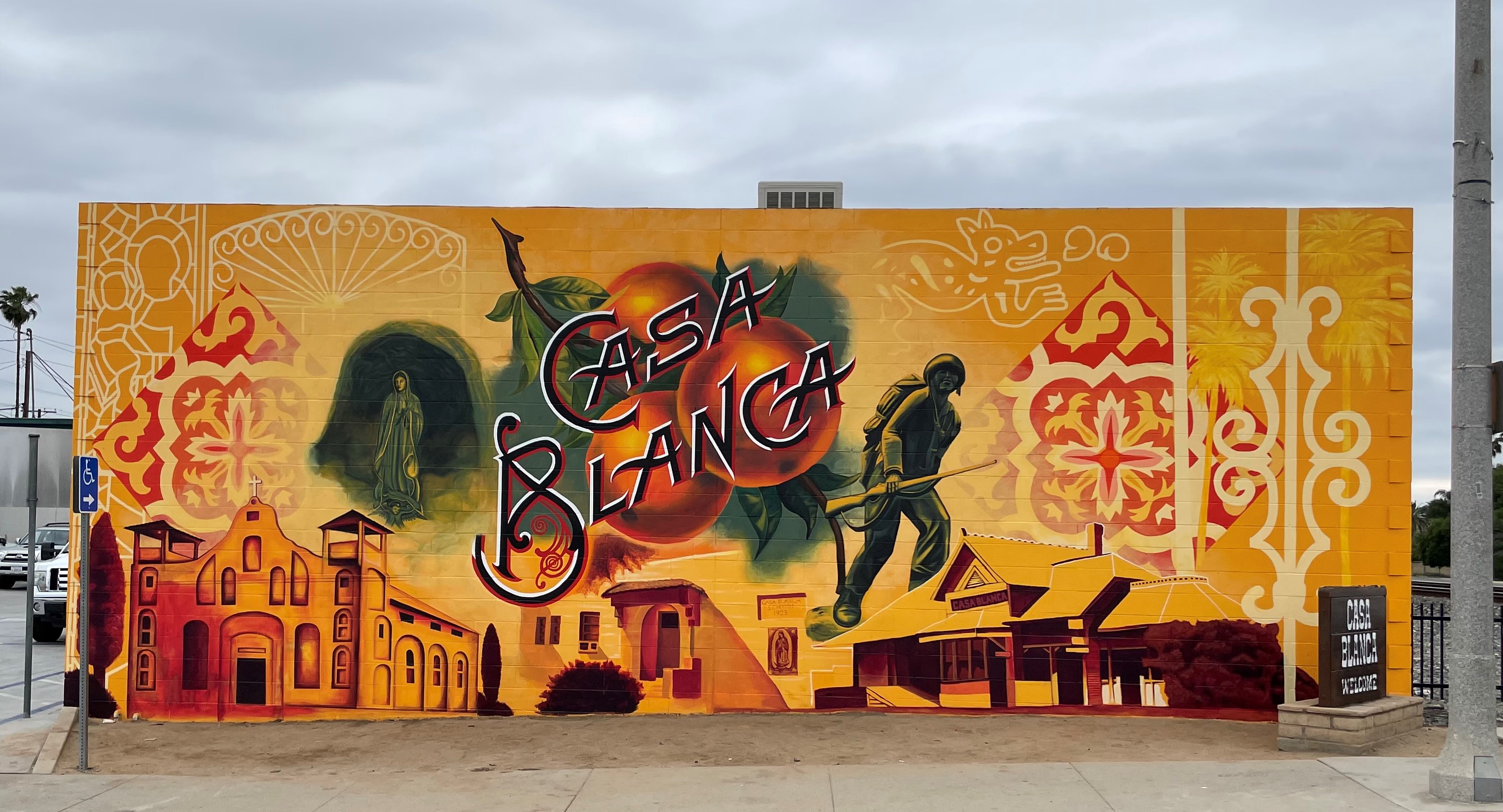This photograph captures a vibrant mural covering the entire side of a building, set against a backdrop of a city street with visible cars. The mural's predominant background is a yellowish-orange hue. Centrally, in elaborate black print, is the text "Casa Blanca," superimposed over realistic depictions of three oranges with green leaves. Below the "Casa Blanca" text, towards the right, stands a Vietnam War soldier, donned in green attire and a helmet, carrying a rifle. To the left of the text is an image of a woman in a black shawl and dress, standing before what appears to be a cave-like entrance.

The lower half of the mural features a series of buildings, painted in black and yellow. On the left is a curvy, church-like structure with a cross atop. In the middle, there's a plain building with a flat roof, arched door, and two windows. To the right, a two-story traditional-looking house faces left, accompanied by a bush. Flanking the mural, intricate diamond patterns in red and white floral designs adorn both sides. Above these patterns, there appears to be a creature resembling a coyote or jackal.

Complementing the mural, a black sign with white lettering reading "Casa Blanca, Welcome" stands on a brick block at the bottom right corner of the wall. This mural is a richly detailed artistic portrayal blending cultural and historical elements, all set amidst an urban environment.